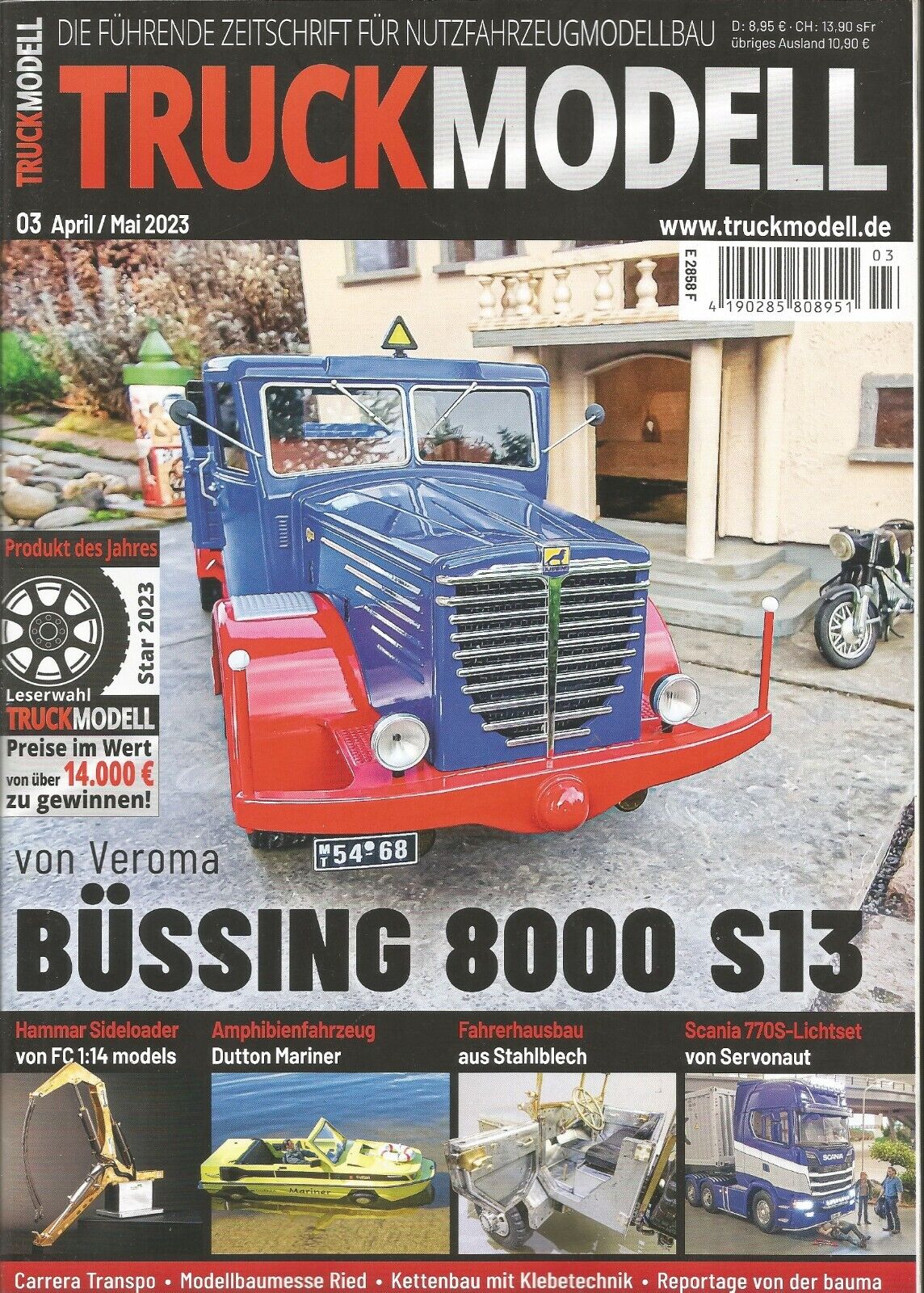The cover of the German magazine "Truck Modell," issue from April 3rd to May 2023, features bold red and white lettering against a black background. Dominating the cover is an angled image of a mostly blue truck with red accents around the wheel wells and round headlights, identified as the Bussing 8000 S13. The truck is parked in front of a European-style mansion driveway. Alongside it, the cover showcases various other truck models such as the FC-14 and Dutton Mariner, depicted in smaller pictures at the bottom. Additional elements include a polished black motorcycle, a barcode, and icons representing different truck parts, with the magazine's URL www.truckmodel.de visible at the top. The report and accompanying text are predominantly in German.